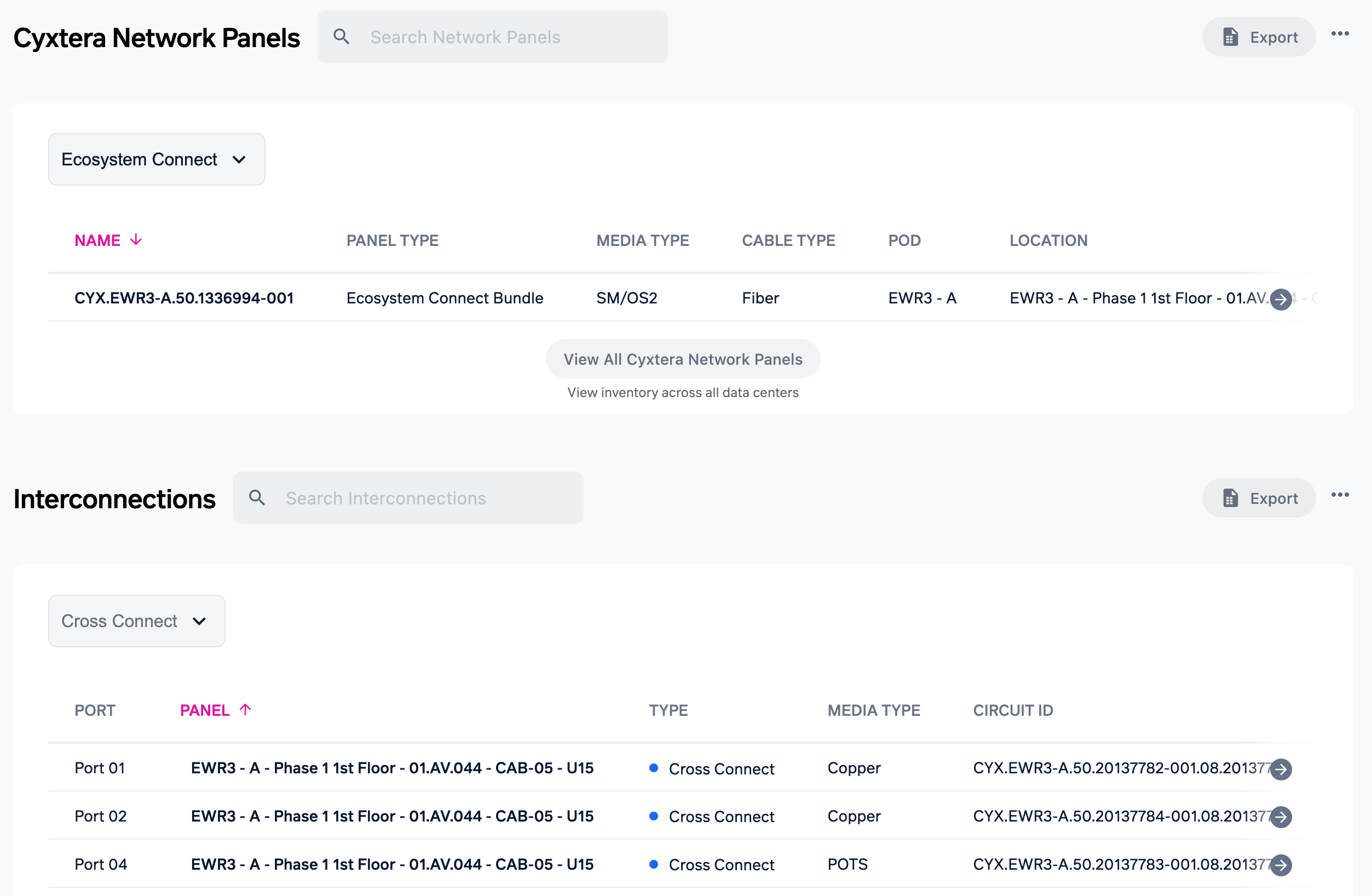This image is a detailed view of a webpage from the website Cyxtera Network Panels. At the top of the page, there's a section with a light gray background, which includes a search bar labeled "Search Network Panels" and an icon of a document next to the word "Export," followed by an ellipsis.

Below this, in a white section, there is a header labeled "Ecosystem Connect" accompanied by a drop-down arrow. Underneath this header, there are columns labeled "Name," "Panel Name," "Media Type," "Cable Type," "POD," and "Location," which likely correspond to various attributes of the network panels. In the center of this section, there's a prominent button labeled "View All Cyxtera Network Panels."

Further down, there's another button labeled "View Inventory Across All Data Centers."

Following this, another gray section appears with the word "Interconnections" and a search bar labeled "Search Interconnections." To the right of this search bar, there's an icon of a document and the word "Export," again followed by an ellipsis.

Finally, another white section appears, featuring a header labeled "Cross-Connect" with a drop-down arrow. Below this header, there is a list of ports categorized under columns labeled "Panel," "Type," "Media Type," and "Circuit ID," listed vertically.